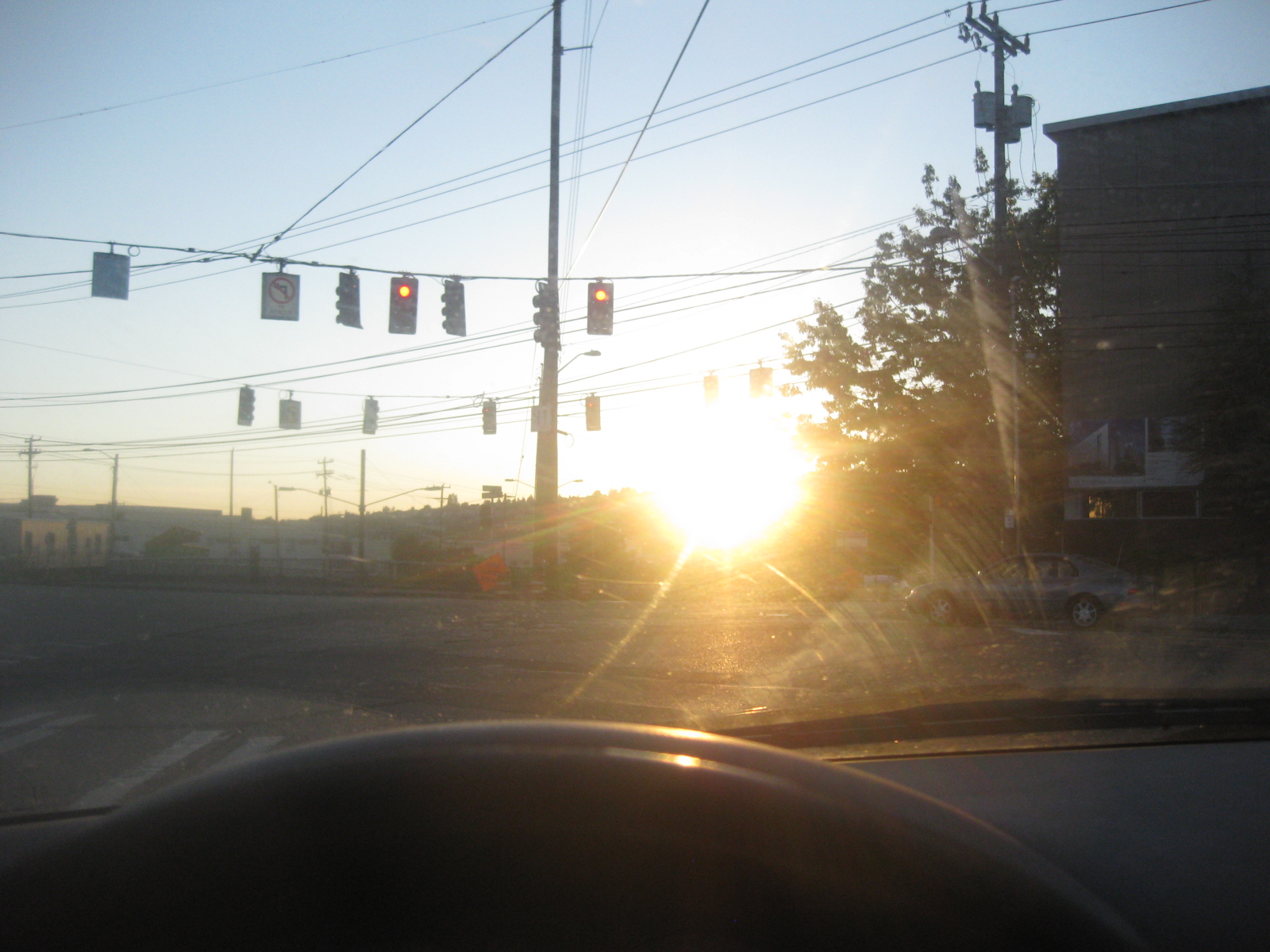Captured from inside a car at a red light, this outdoor photograph offers a unique perspective through the windshield. The scene includes the curved top of the dashboard and the upper section of the steering wheel. Illuminating the setting is a brilliant sunrise, low in the sky and nearly blinding in its intensity. The background features a residential neighborhood with several houses and a building on the corner that resembles a house. In front of this building, a car is parked on the street. Multiple traffic lights are suspended from overhead wires, accompanied by a telephone pole adding to the urban landscape. The sun appears over a slightly hilly region in the distance, casting light on numerous buildings in the background. The street below includes a visible crosswalk, and within the vehicle, only a snippet of the dashboard and a windshield wiper are discernible.